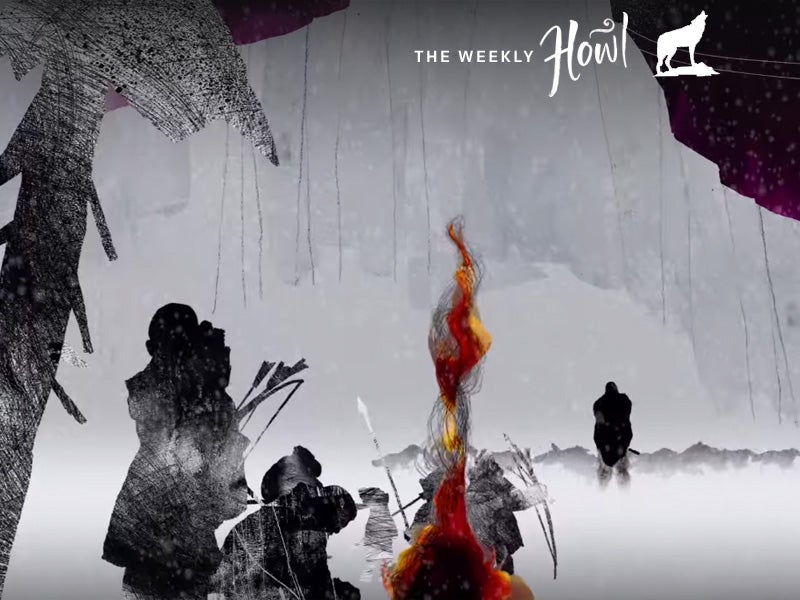This digital art piece, reminiscent of an abstract collage, uses predominantly gray tones to create a dramatic contrast with a vivid central flame of dark browns, reds, golds, and whites, with gray smoke intermingling above it, somewhat hastily hand-drawn. Surrounding this central fire are black, white, and gray silhouettes of figures, some wielding bows and arrows and others brandishing spears, reminiscent of cavemen or Native American hunters. To the left of the flame, a tree stands starkly against the background, its silhouette stretching from the bottom left towards the top left. In the far right, a figure draped in a thick outer garment looks off into a misty, gray expanse, suggesting a distant, snowy landscape or a cliff. Above this enigmatic scene, in the top right corner, a logo in flowy, cursive text reads "The Weekly Howl," accompanied by a small white outline of a howling wolf, adding an ethereal touch to this hauntingly beautiful composition.